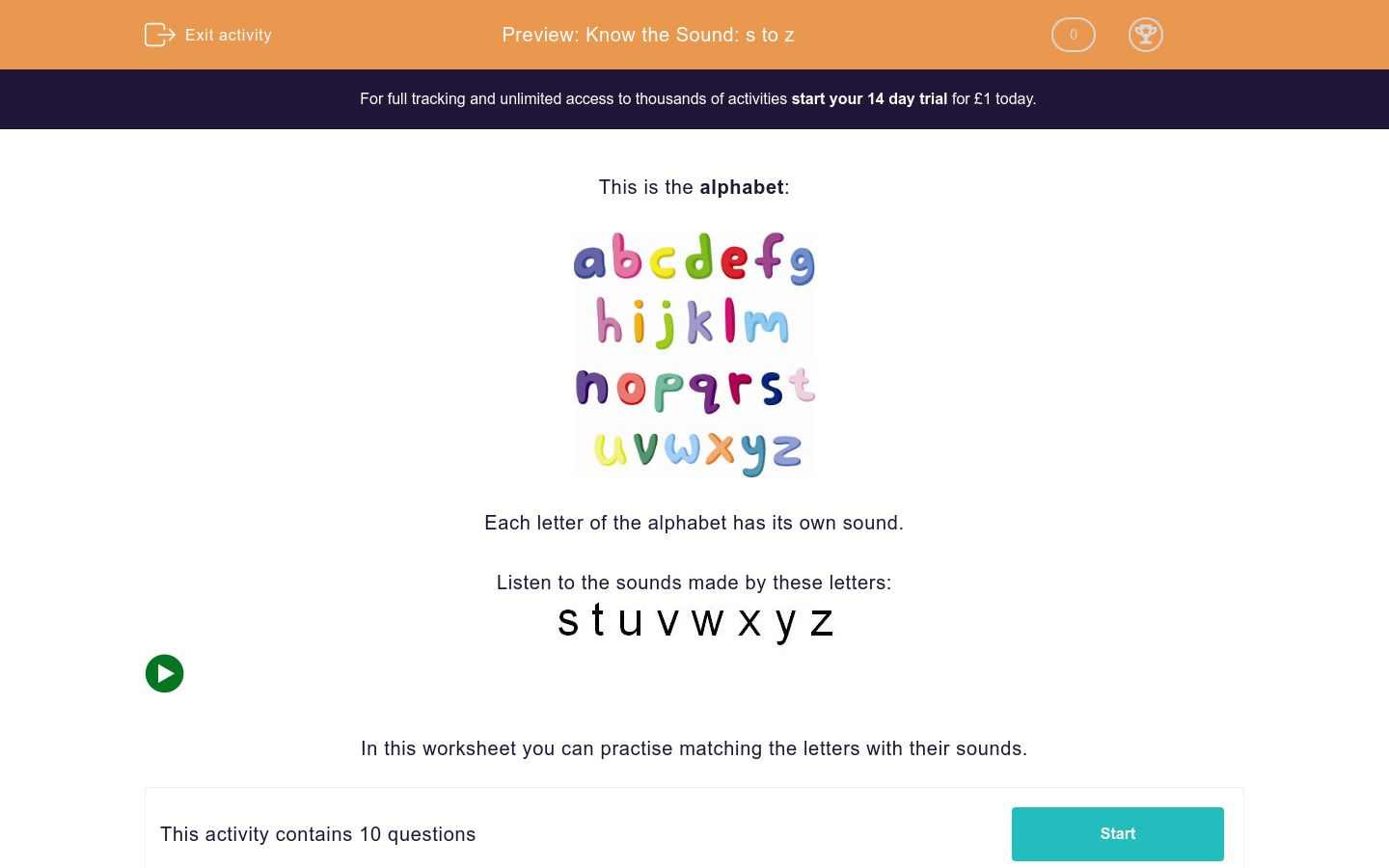This is a detailed, cleaned-up caption for the described image:

---

A screenshot from an educational webpage is presented. At the top of the page, there is an orange border with centered white text that reads, "Preview: Note the sound, S to Z." To the left of this text, there is an "Exit Activity" button, and to the right, there are two icons: one with a circular zero and the other featuring a trophy symbol, indicating awards. Below this, a black background section contains white text promoting a 14-day trial for £1, stating, "For full tracking and unlimited access to thousands of activities, start your 14-day trial for £1 today."

The main content area beneath has a predominantly white background. Centrally displayed is the alphabet in a playful, childlike font with bright colors such as pinks, yellows, greens, lime greens, and light blues. The alphabet is divided across four lines: A to G, H to M, N to T, and U to Z. Each letter is lowercase and individually colored. Accompanying text explains that each letter has its own sound and instructs users to listen to the sounds made by these letters.

Below the alphabet, in smaller black text, it reads, "In this worksheet, you can practice matching the letters with their sounds." On the left side of this section, there is a green button with a triangle icon, indicating a video thumbnail that can be clicked. Additional text is beneath this button, though it is not specified in detail.

At the very bottom of the page is a prominent green button with white text that says "Start."

---

This detailed caption provides a clear and organized description of the webpage screenshot for further clarity.